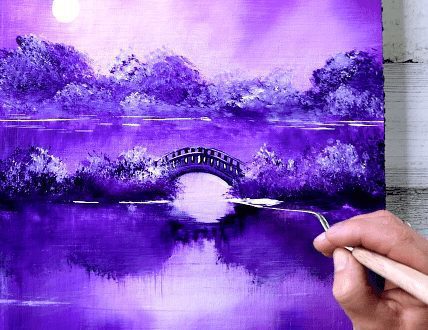The photograph captures an artist meticulously applying finishing touches to a serene landscape painting, primarily rendered in various shades of purple and lavender. Taking up most of the image, the square canvas showcases an arched Victorian-style bridge with railings, centrally positioned over a body of still water, which mirrors the sky and surrounding bushes and trees. The backdrop includes a subtle, hazy full moon or sun in the upper left, lending a tranquil ambiance to the scene. The artist's Caucasian hand, possibly male, holding a metal-topped painting tool with a beige wooden handle, is visible in the bottom right corner, highlighting their engagement with the artwork. The painting rests on a flat, white surface, while on the far right, the background features a wall of white-painted wooden boards. The intricate use of purple hues and delicate white accents effectively brings to life the reflective water, lush foliage, and peaceful sky, creating a traditional yet captivating depiction of nature.